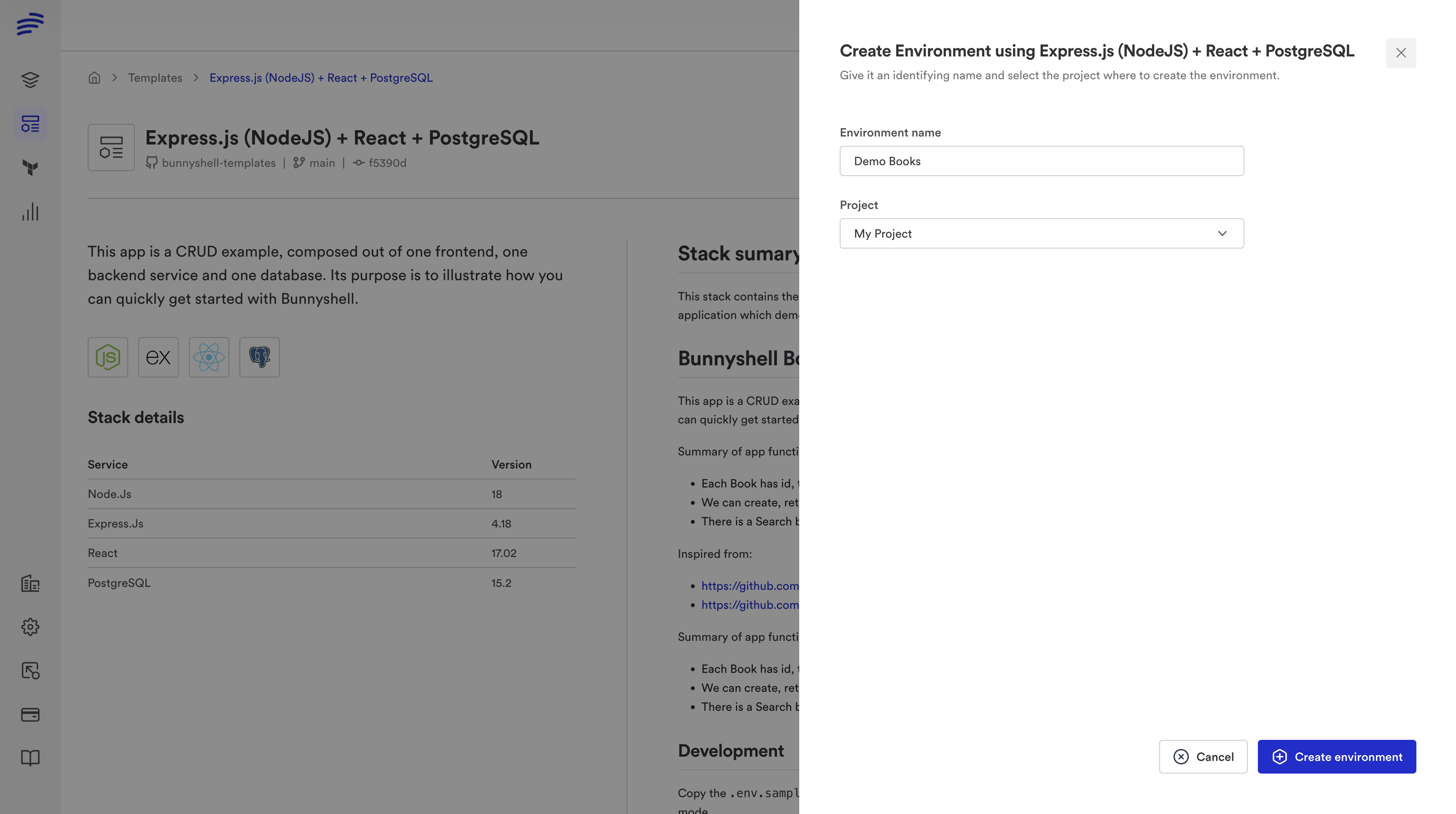This screenshot showcases a white screen from an unspecified device, potentially a mobile device or a PC. At the top of the screen, the title "Express.js" is prominently displayed, followed by "Node.js" in parentheses, and further coupled with "React" and "PostgreSQL." Below this title, a detailed description explains that the application is a CRUD (Create, Read, Update, Delete) example, consisting of a frontend, a backend service, and a database. The primary purpose of this app is to demonstrate how users can quickly begin utilizing BunnyShell. The right-hand side of the screen contains additional information about the stack summary, but this portion is unfortunately cut off and unreadable. This screen appears to pertain to the realm of computer programming or coding, likely part of a programming application or tool.